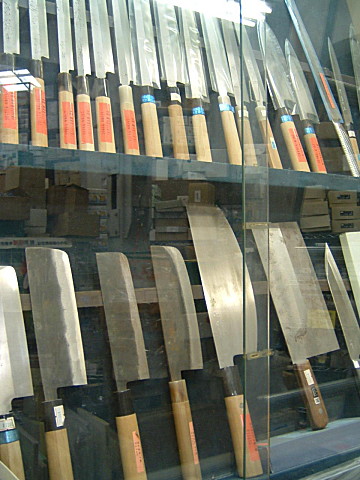The image depicts a glass display case with two blue-painted shelves inside, likely located in a store. The top shelf features a variety of carving knives, all with wooden handles and some adorned with blue, orange, or white price tags. These knives have thinner, pointed blades, some resembling straight razors used in barbershops. In contrast, the bottom shelf showcases butcher knives and large cleavers, characterized by their broad, rectangular blades and also featuring wooden handles with similar price tags. The display case has sliding glass doors, evident from the reflections and the overlapping panes, indicating a retail setting, possibly a specialized knife shop.